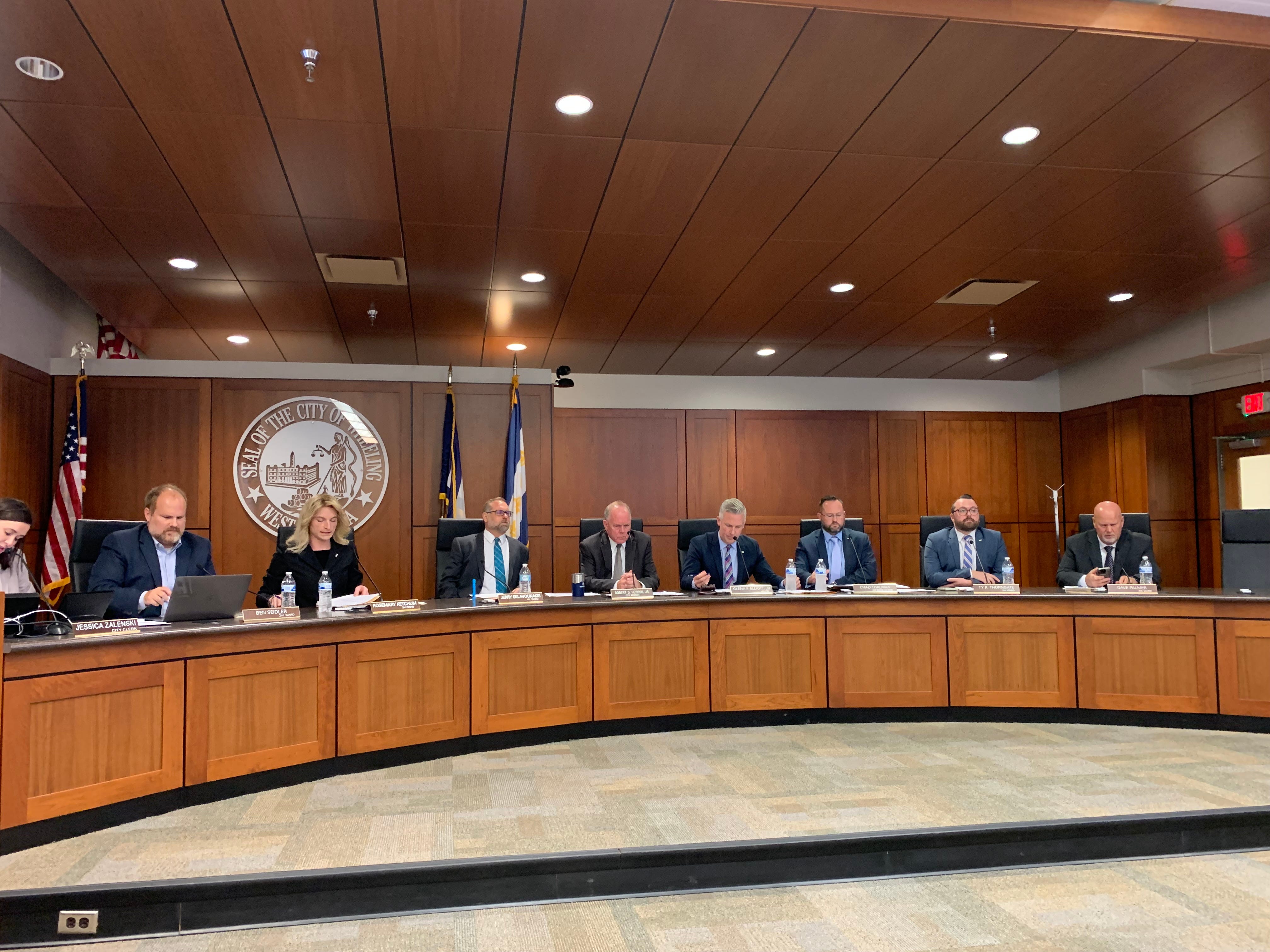The photograph captures the interior of a government-style building in the United States, likely a city council chamber or similar democratic setting. The room is distinctly professional, featuring wooden-clad walls and a dark wooden ceiling with spotlights that provide ample lighting, albeit causing a slight distortion on the seal. Prominently displayed on the back wall is the seal of the city, though its full name is obscured by reflections and an individual standing in front. The visible text reads "Seal of the City of West [something ending in 'A']." 

To the left of the seal, an American flag stands tall, accompanied by two other flags close by. The room's ambiance is further characterized by brown paneling on both the desk and walls. In the foreground, a large, oval-shaped desk faces a presumed audience, with about nine professionally dressed individuals seated around it, leaving one chair empty on the right. These individuals appear to be elected officials or judges, given the name plaques, water bottles, and paperwork in front of them. Among these officials, two are women and the rest older men, with one notably bald. One of the men is actively using a computer.

The floor in front of the officials is carpeted, stepping down to another carpeted area, adding layers to the room's structured layout. Overall, the photograph conveys a formal, authoritative atmosphere typical of a governmental assembly or judicial proceeding.